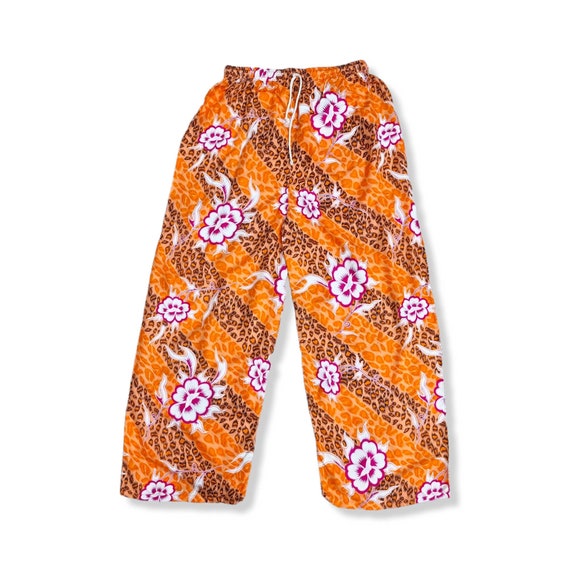This image depicts a pair of loose-fitting cotton trousers set against a plain white background with subtle gray shadows on the right side and bottom of each leg. The trousers feature an elastic waistband equipped with white drawstrings, which appear crinkled or wrinkled, indicating their stretchability.

The fabric of the trousers showcases a distinct, repeating pattern. The base color is a light tan to light orange hue adorned with darker orange leopard print, characterized by oblong circles and dots that create a lively, animal-inspired design. Adding to this are larger stripes with similar leopard print in darker shades of orange. Interspersed within this pattern are large white flowers outlined in pink or purple, with purple centers and leaves featuring purple tinges, creating a dynamic and eye-catching design that covers the entire pair of pants. The detailed and vibrant pattern flows diagonally from the upper left to the lower right of the trousers, adding a visually engaging element to the garment.